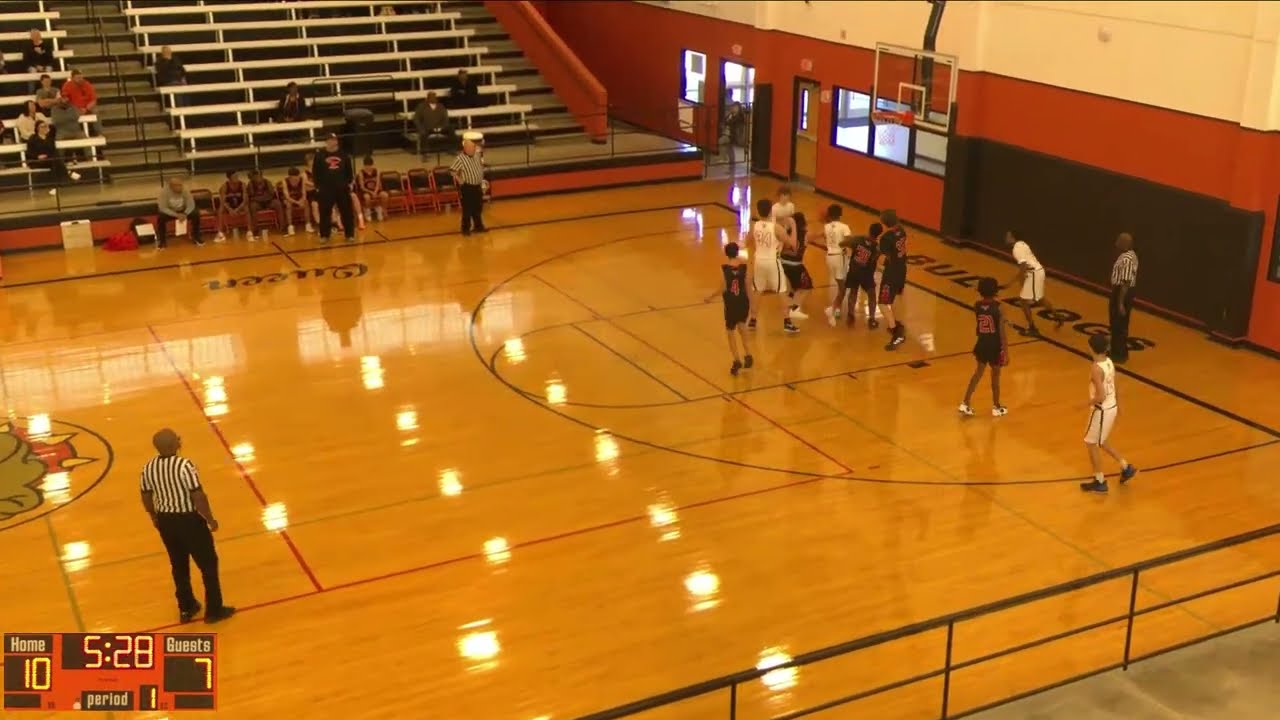In this high school basketball game, a digital photograph captures the intense action on an indoor court with a gleaming wood floor, so polished that the ceiling lights reflect vividly off its surface. The focus is on the two teams competing—one in black uniforms (black tops and shorts) and the other in white (white tops and shorts). The game is five minutes and 28 seconds into the first period, with the home team leading 10 to 7, as displayed prominently on a scoreboard in the bottom left corner. The left side of the image features a referee in a traditional white and black striped shirt with black pants, closely monitoring the play. In the top left, sparse spectators are seated in the stands, just above the benches where extra players sit, while another referee can be seen on the right side of the image, overseeing the players who are engaged in action near the hoop. The scene is rich with details, from the visible basketball hoop, net, and backboard to the glimpse of doors and windows in the background, and even the school team name, "Bulldogs," marking the home advantage.